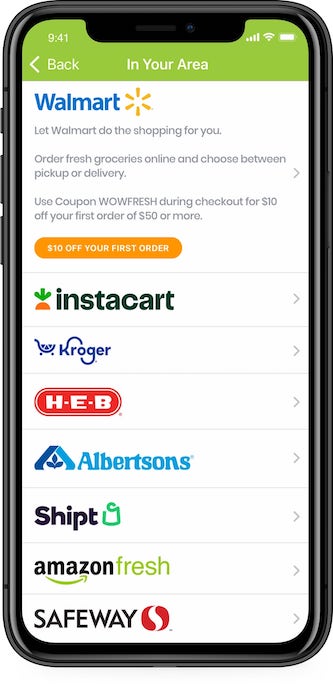The image displayed on a cell phone screen showcases a detailed interface. The top portion of the screen is shaded in green. In the upper left-hand corner, the time is displayed as 9:41 AM. Beneath the time, there is a white left-pointing arrow accompanied by the word "Back." Centered within the green-shaded area is the text "In your area." In the top right corner of this green section, the Wi-Fi signal, battery life, and cellular signal icons are visible.

Below the green header, the majority of the cell phone screen is white. In the top left corner of this white section, there is a blue "Walmart" logo alongside a small sunshine emblem. Underneath the logo, a message in dark gray text reads: "Let Walmart do the shopping for you. Order fresh groceries online and choose between pickup or delivery. Use coupon WowFresh during checkout for $10 off your first order of $50 or more." 

Below this description, an orange bubble contains white text that says, "$10 off your first order." A gray line divides this section from the list beneath.

Subsequently, a list of grocery service options is presented with black text and each brand name followed by a small, gray right-pointing arrow indicating further details. The options listed are:

- Instacart
- Kroger (in blue text)
- H-E-B
- Albertsons
- Shipt
- Amazon Fresh
- Safeway